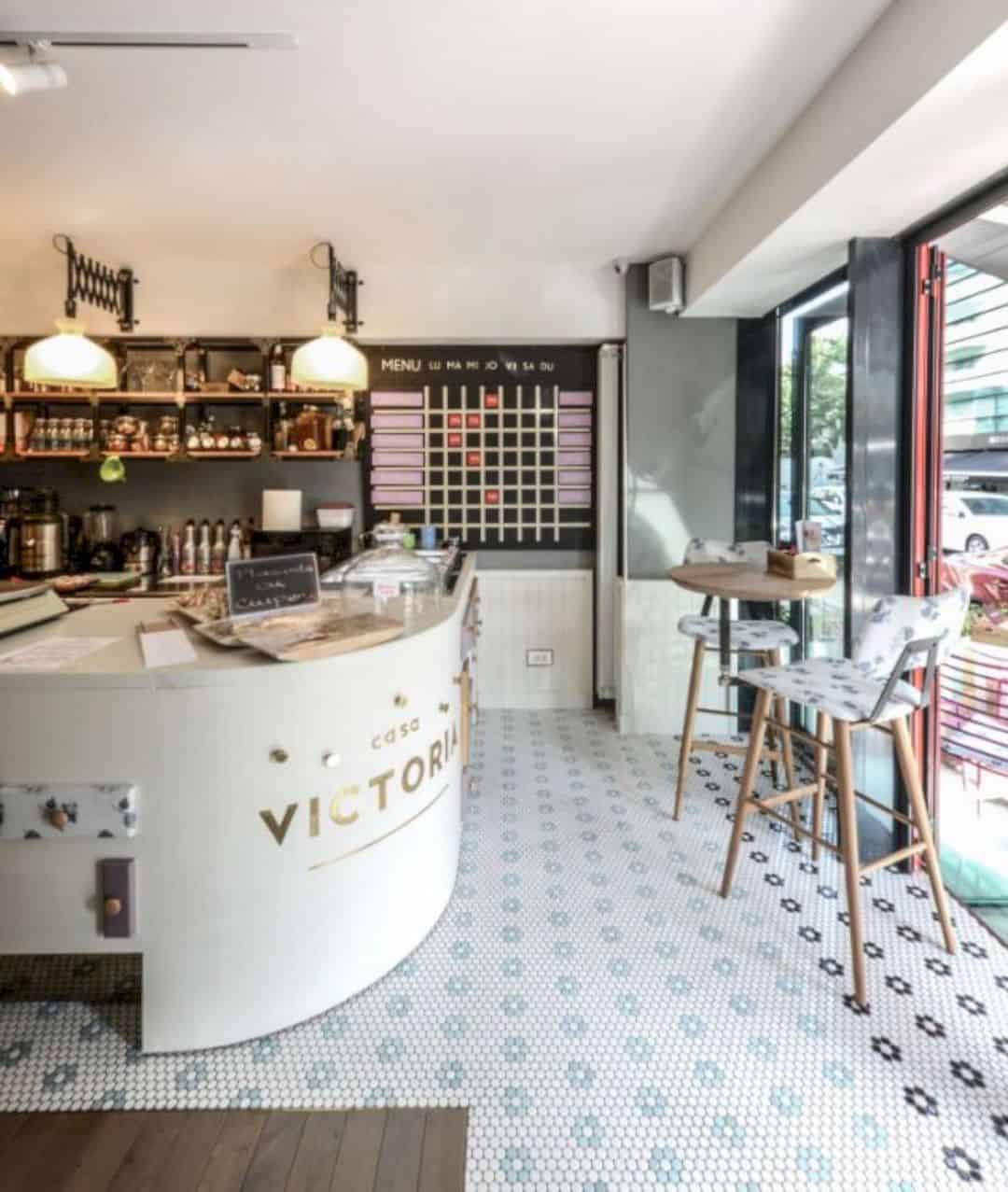This image captures the inviting interior of what appears to be a cozy coffee shop named "Casa Victoria." On the left side of the picture, the shop's counter prominently displays the establishment's name. Just above the counter, a charming chalkboard warmly welcomes customers. Behind the counter, a menu board designed to look like a game board features a grid pattern with little red dots, adding a playful touch to the decor. 

In the top left corner, shelves adorned with various spices give the space a homely feel. Two brightly lit, wall-mounted lights illuminate the room, casting a warm and welcoming glow. On the right side, a small coffee table accompanied by two barstool chairs with unique patterns offers a cozy spot for patrons. The floor boasts an interesting linoleum finish, adorned with circle patterns resembling roses.

On the far right side of the image, large glass windows reveal a glimpse of the bustling city life outside, with cars driving up and down the streets. This small coffee shop, with its distinctive decor and inviting atmosphere, stands as a unique retreat within the urban landscape.